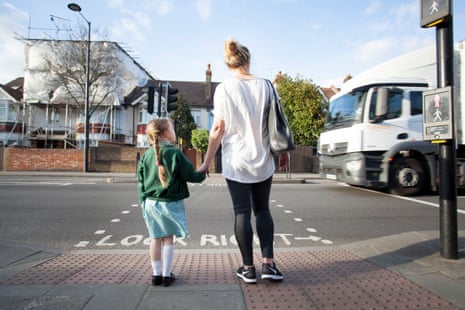A woman and her young daughter are standing stationary on a sidewalk at a crosswalk, waiting to safely cross the street on a bright, sunny day. The woman, who appears to be preparing for a gym visit, is outfitted in a white t-shirt over black joggers or yoga pants, with black sneakers and a purse slung over her shoulder. Her blonde hair is tied back in a ponytail. She holds the hand of her daughter, a school-age girl of about six or seven years old, who is dressed in a green sweater or hoodie, a blue skirt, long white socks, and black shoes. The girl's hair is long and braided, matching her mother’s blonde tresses. They are both looking at a large white truck that is approaching the intersection. In the background, a few trees and a building, possibly residential or industrial, are visible against a light blue sky with wispy clouds. The crosswalk in front of them is marked with the words "LOOK RIGHT" painted on the road, and there is a pedestrian walk sign next to them as they wait to yield to the oncoming traffic.